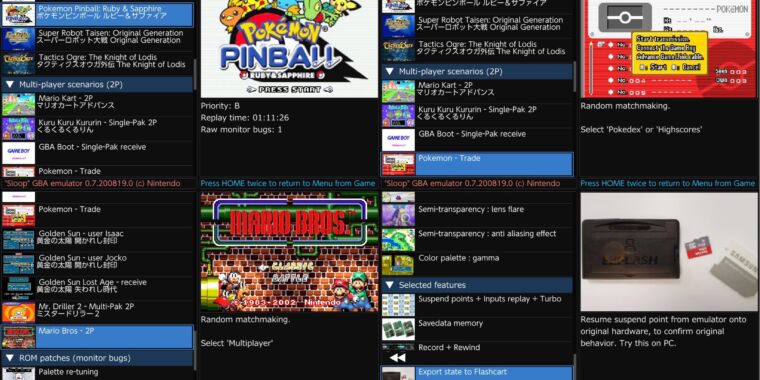A vibrant and highly content-packed web page is divided into four equal sections. The left-most pane features numerous thumbnail images accompanied by text, predominantly in Chinese characters with sparse English phrases interspersed. The second pane showcases the cover image and title for "Pokemon Pinball," followed by annotated details such as "Priority B," "Replay Time: 01:11:26," and "Raw Monitor Bugs: 1." Below this, another section highlights an image from the "Mario Bros" video game, with instructions labeled "Random Matchmaking" and "Select Multiplayer." The third pane mirrors the first, with a mix of images and bilingual text. The fourth and final pane on the right displays a Pokemon Pokedex interface with menu options labeled "Random Matchmaking," "Select Pokedex," and "High Scores." Beneath these menu options, there is an image that appears to depict either a flash or SIM card.